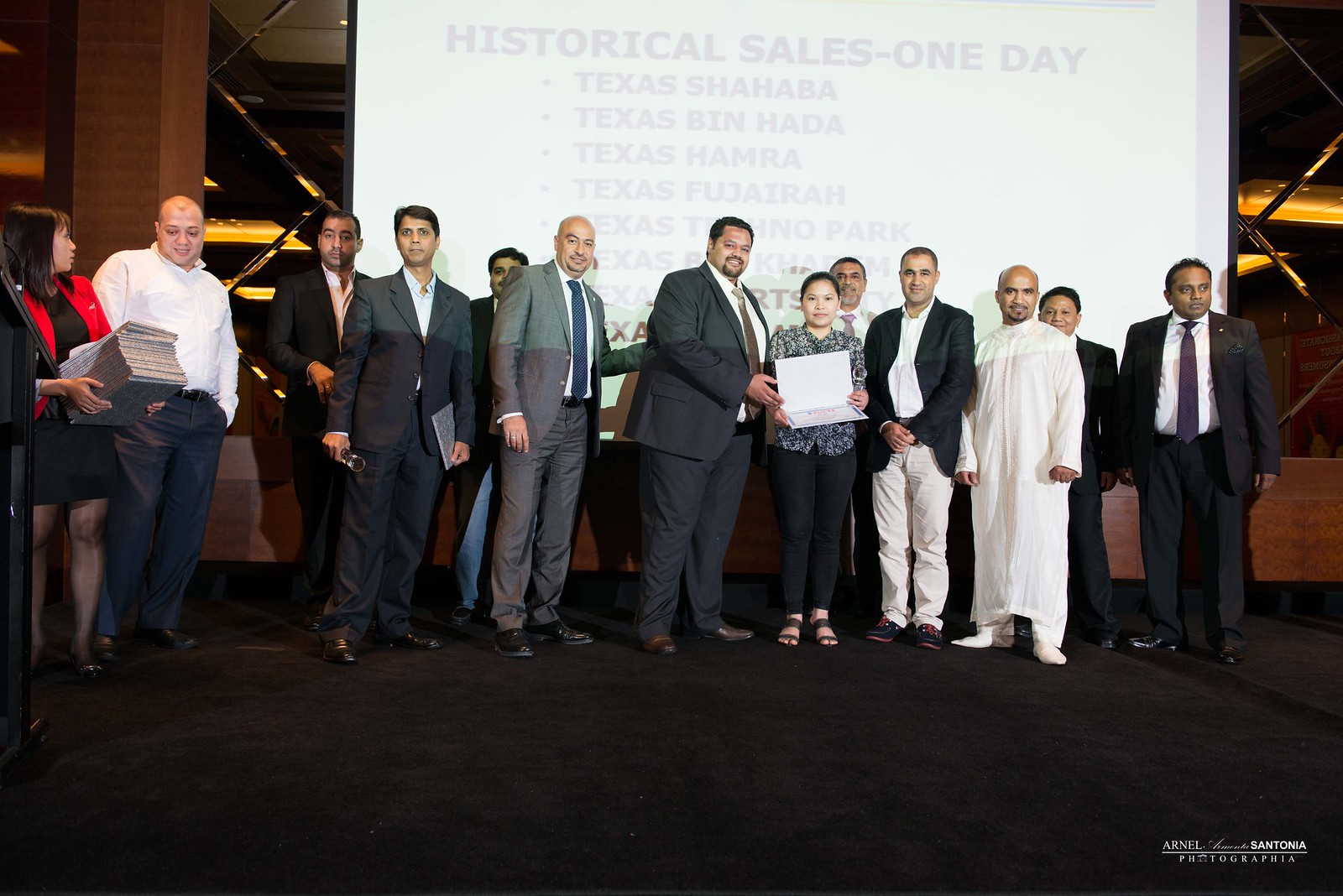The photograph showcases approximately 15 people, both men and women, posing together in an indoor setting. The group, many of whom are dressed in suits and ties, stands on a dark-colored carpet. Central to the image is a woman holding an open certificate, though the details of the certificate are illegible from a distance. To her left, a large man assists her by holding the certificate with his right hand. On the far left, another woman stands behind a podium with several books in her hand. Behind the group, a substantial white projector screen displays the text "Historical Sales One Day," followed by partially obscured text listing various Texas locations: Shahaba, Benhada, Hamra, and Fuhajara. In the bottom right corner of the image, there is a watermark from the photographer, Arnel Sentonia Fotografia.